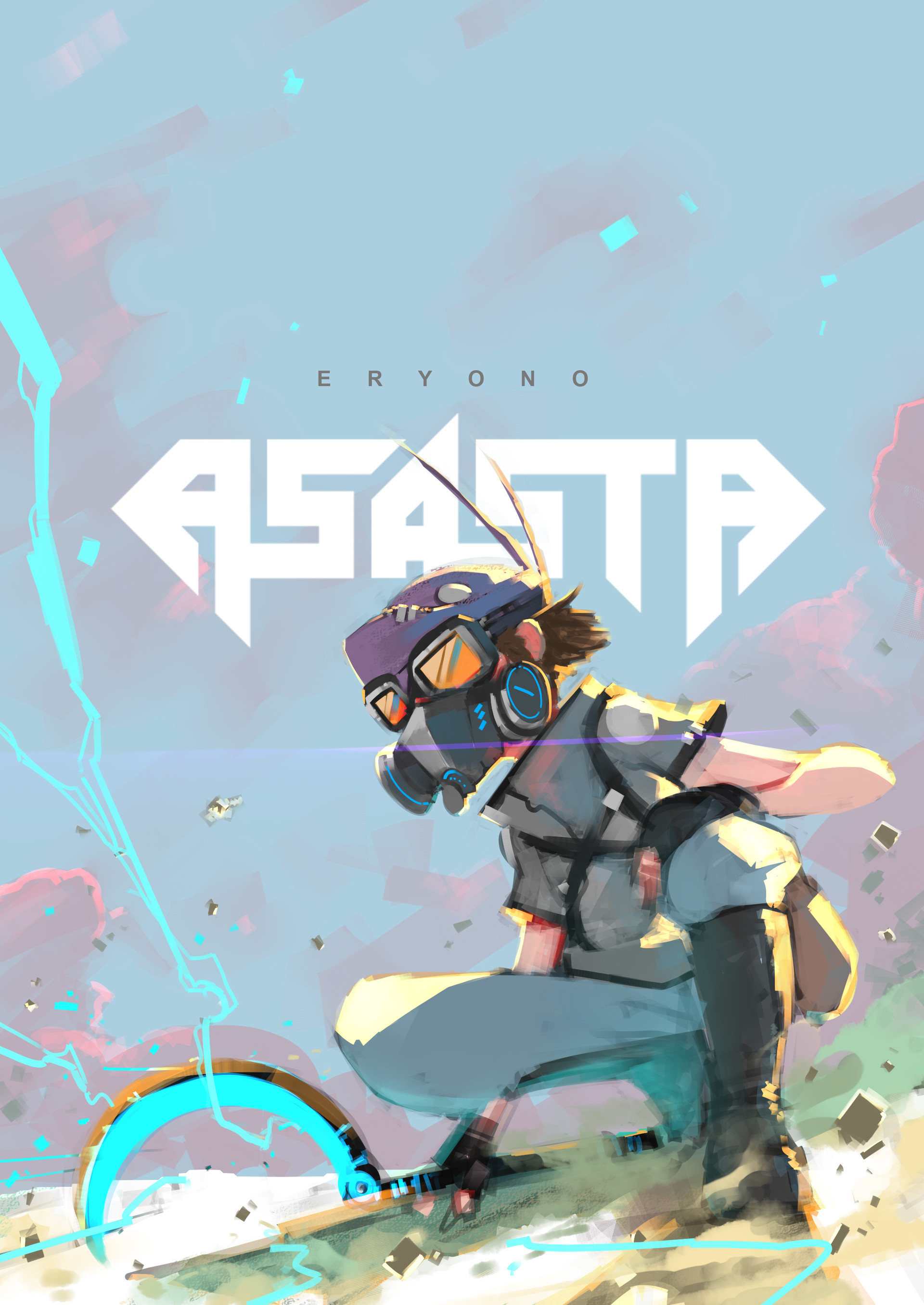The image is a detailed digital illustration, likely a poster or artwork with a light blue background accented by faint smudges of red and pink clouds. The title at the top of the image reads "Eriyono" in black text, and underneath it, "Asasta" is written in a spiffy, angular white font shaped like a diamond heart. Central to the image is a character resembling a child wearing a distinctive gas mask with orange-tinted, square lenses encased in silver frames. The mask includes a ventilator piece with two air vents, giving it an almost futuristic look. The character is dressed in a light gray short-sleeve shirt with black straps crossing the chest, white or gray pants, and knee-length black boots. They are kneeling or squatting on what appears to be rocky terrain, possibly grass or sand, and are holding a striking blue sickle with a yellowish outline electrified with turquoise lightning. The detailed rendering and unique elements suggest the image may be inspired by video game aesthetics.